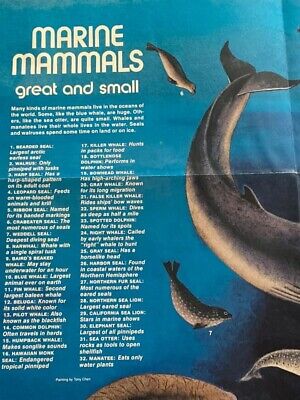This image features a page from an illustrated book or magazine on marine mammals. The background is a turquoise blue, and the top left corner prominently displays the title "Marine Mammals Great and Small" in white text. Below this title, there's a small, unreadable paragraph likely describing the content of the book or article, and beneath that is a numbered list ranging from 1 to 32, categorizing various marine animals. The right side of the page showcases images of different marine mammals, including several seals and the partially visible tail end of a finned animal, possibly a whale, with the front part cut off. At the bottom of the page, there is a brown, rounded image that appears to be another marine animal, though its specific identity is unclear.